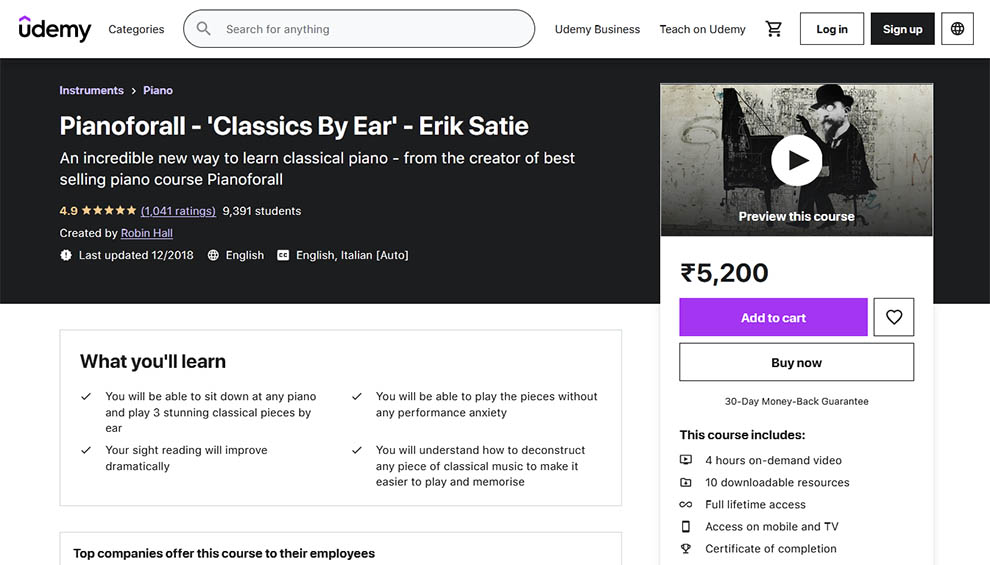A screenshot of the Udemy homepage features prominently. The distinctive Udemy logo is displayed at the top left, with a unique purple emblem atop the 'U' and the name 'Udemy' spelled out in lowercase bold black letters. To the right of the logo, a navigation menu appears with smaller font options like 'Categories,' followed by a search bar. Adjacent to this are links for 'Udemy Business,' 'Teach on Udemy,' a shopping cart icon showing it's empty, and options to log in or sign up. There’s also an icon for accessing the user’s profile.

Below the main navigation, a gray banner highlights various piano courses under the category 'Instruments, Piano.' The phrase 'Instruments, Piano' is displayed in violet, while the specific course name 'Piano for All, Classics by Ear, Eric Satie' is bolded in white. Directly beneath this, a promotional text reads: "An incredible new way to learn classical piano from the creator of the best-selling piano course, Piano for All." The course boasts a near-perfect 4.9-star rating and has been taken by almost 9,000 students. A thumbnail image of the course appears to the side, with purchasing options clearly stated – the course is available for 5,200 units of an unspecified currency. Buttons to 'Add to Cart' and 'Buy Now' are provided, along with details on what the course covers.